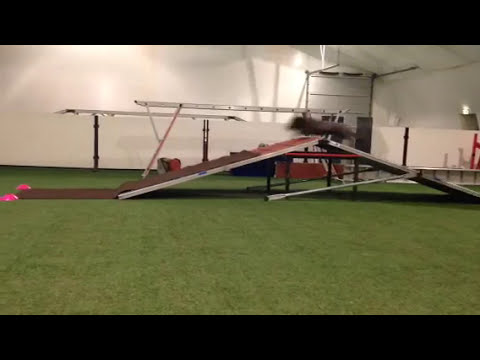The image depicts a large, indoor dog training center or competition setup, characterized by white walls and ceiling. Black borders frame the top and bottom of the screen, focusing attention on a central dog agility course. The foreground features a ramp which the dark-colored dog, captured mid-motion at the highest point, is rapidly navigating. The ramp is covered in brown carpeting secured by pink stops, with green fake grass spread beneath it. The backdrop includes various metallic structures, possibly hurdles or ladders, which serve as additional obstacles in the course. The overall scene is set within what appears to be a spacious gymnasium-like environment.